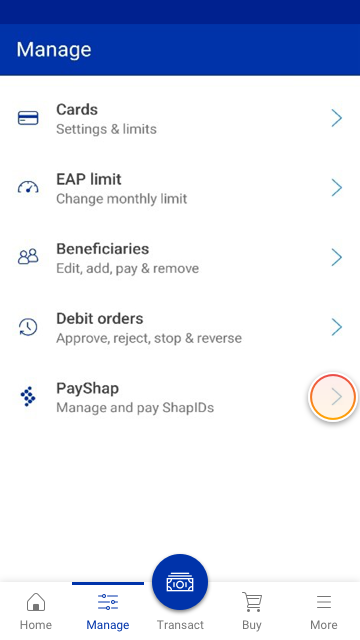A rectangular screenshot depicts a cell phone screen with a user interface focused on management features. In the upper left corner, the word "Manage" is displayed in white text against a dual-tone rectangular bar featuring shades of blue. Below this header, the left side of the screen lists several management options including "Cards," "EAP Limit," "Beneficiaries," "Debit Orders," and "Payshap." Each option is accompanied by an icon. Specifically, the "Payshap" option has a distinct circular icon outlined in a gradient of red and yellow, filled with a light peach background, and featuring a right-facing light gray caret arrow.

At the bottom, a navigation menu is visible, displaying icons for "Home," "Manage," "Transact," "Buy," and "More." The "Transact" button stands out as a large circular icon with a dark blue background adorned with a white stack of dollar bills. The "Manage" button to the left of "Transact" is highlighted, indicated by a horizontal blue bar above it, and both its text and icon are in dark blue, signifying it as the currently selected option.